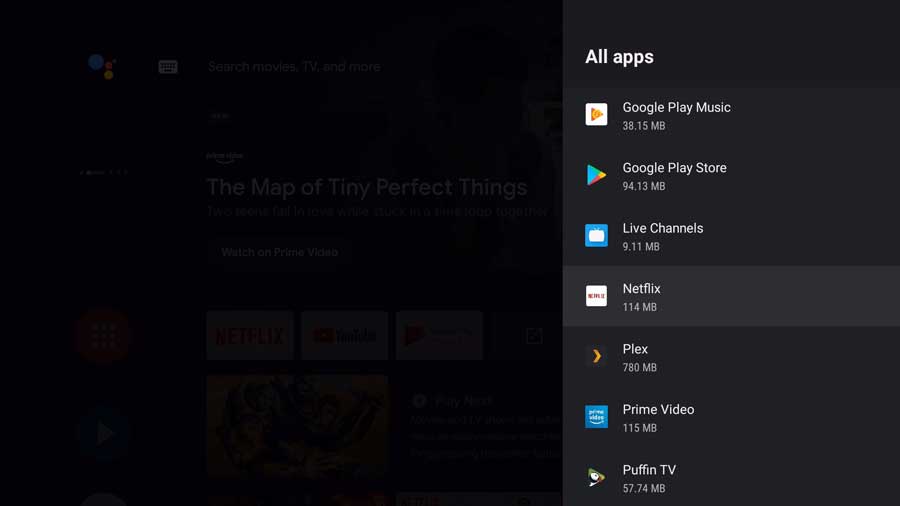Screenshot of a smart TV interface featuring a black background with a transparent overlay on the left and a detailed app menu on the right. The menu is titled "All Apps" in white text and lists several applications with their respective storage usage, each accompanied by the app's logo. The applications listed are Google Play Music (38.15 MB), Google Play Store (94.13 MB), Live Channels (9.11 MB), Netflix (1.14 MB, currently highlighted), Plex (780 MB), Prime Video (115 MB), and Puffin TV (57.74 MB). On the left side of the screen, through the dark overlay, there is faint text promoting "The Map of Tiny Perfect Things" available to watch on Prime Video, alongside what appears to be a user profile section faintly visible in the background.